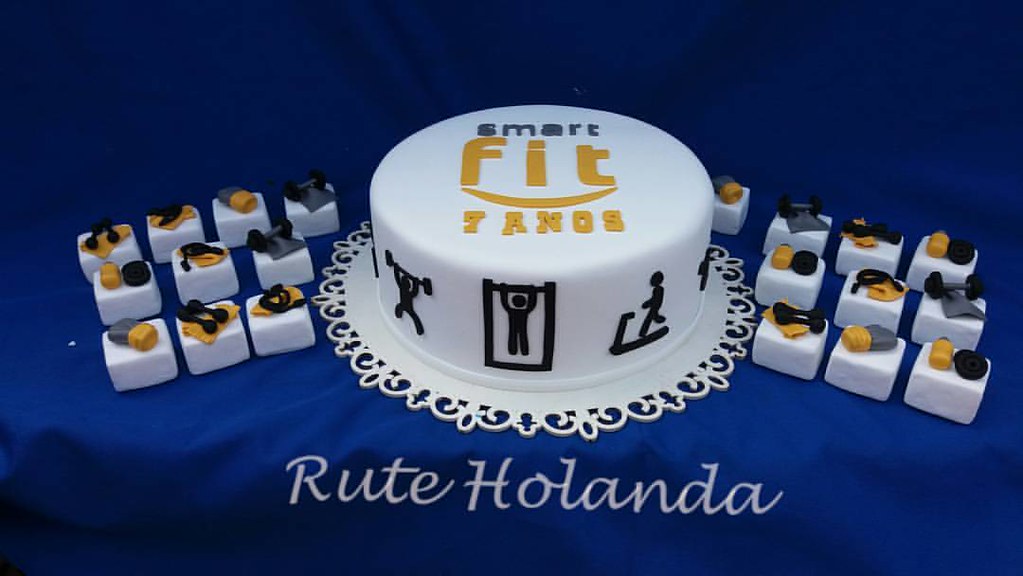The image depicts a large round white cake centered against a dark blue background. The cake features both black and gold lettering, with the words "Smart" in black and "Fit Janos" in gold. The middle-bottom portion of the cake is adorned with a fancy loop. Surrounding the cake are twenty small square cakes, ten on each side, each topped with gray, yellow, and black decorations that resemble gym equipment. The cake itself also has symbols of various exercises, including a figure doing pull-ups, another running on a treadmill, and one lifting a barbell. At the bottom of the image, on the blue tablecloth, the name "Root Hollanda" is written.